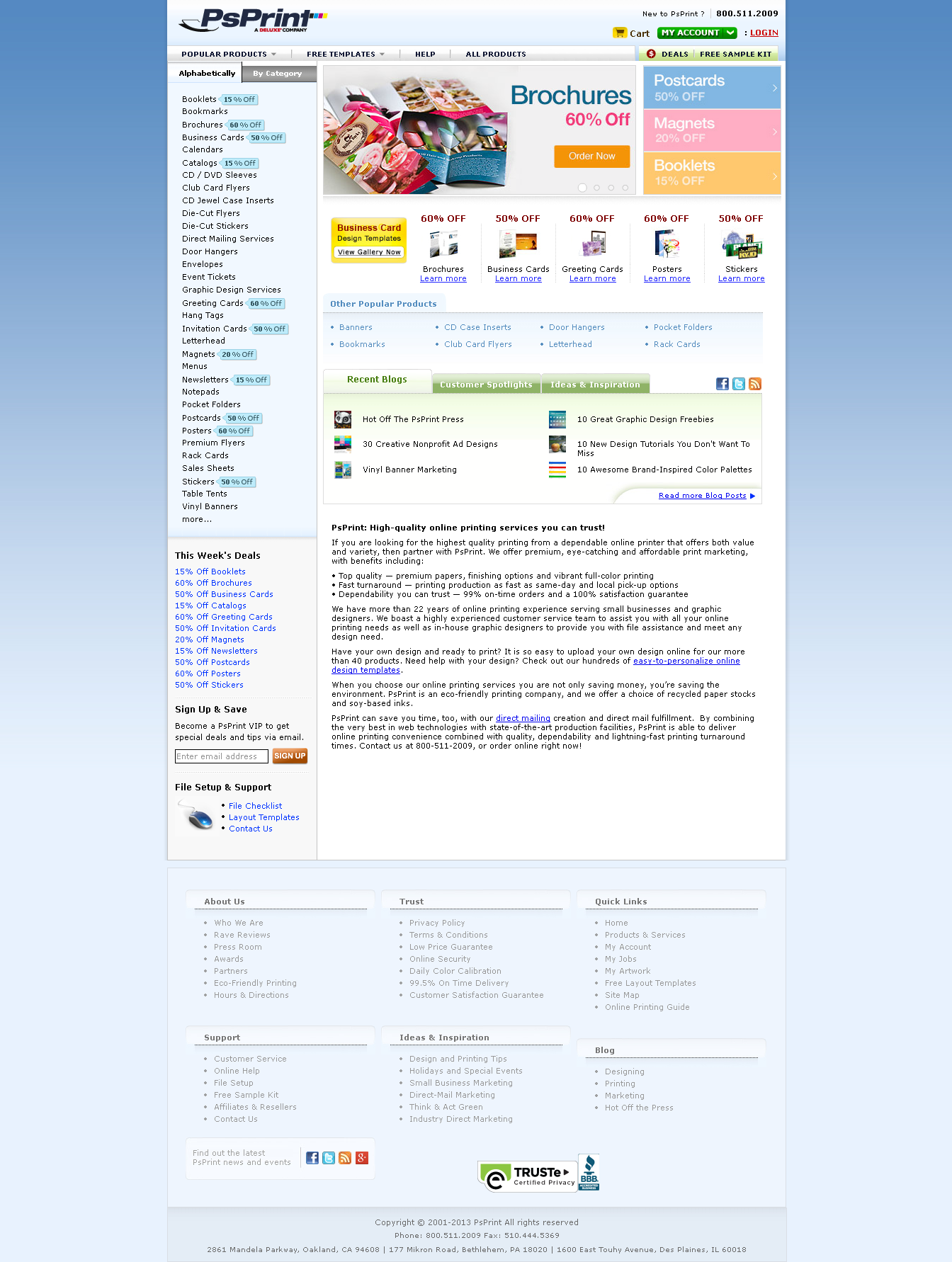Screenshot of the PS Print website. At the top, the PS Print logo is prominently displayed in a dark blue font. Below the logo, on the left-hand side, a menu features several lines of black text followed by a list of links highlighted in blue. Centrally positioned on the page is an image showcasing various brochures, with the word "brochures" written in blue text and "60% off" noted in red beneath it. Surrounding this central image are clickable items leading to similar products. Further down the page, a set of social media icons – including Facebook and YouTube – are available for interaction. The page also contains approximately five paragraphs of detailed black text, ending with a blank white section at the bottom.